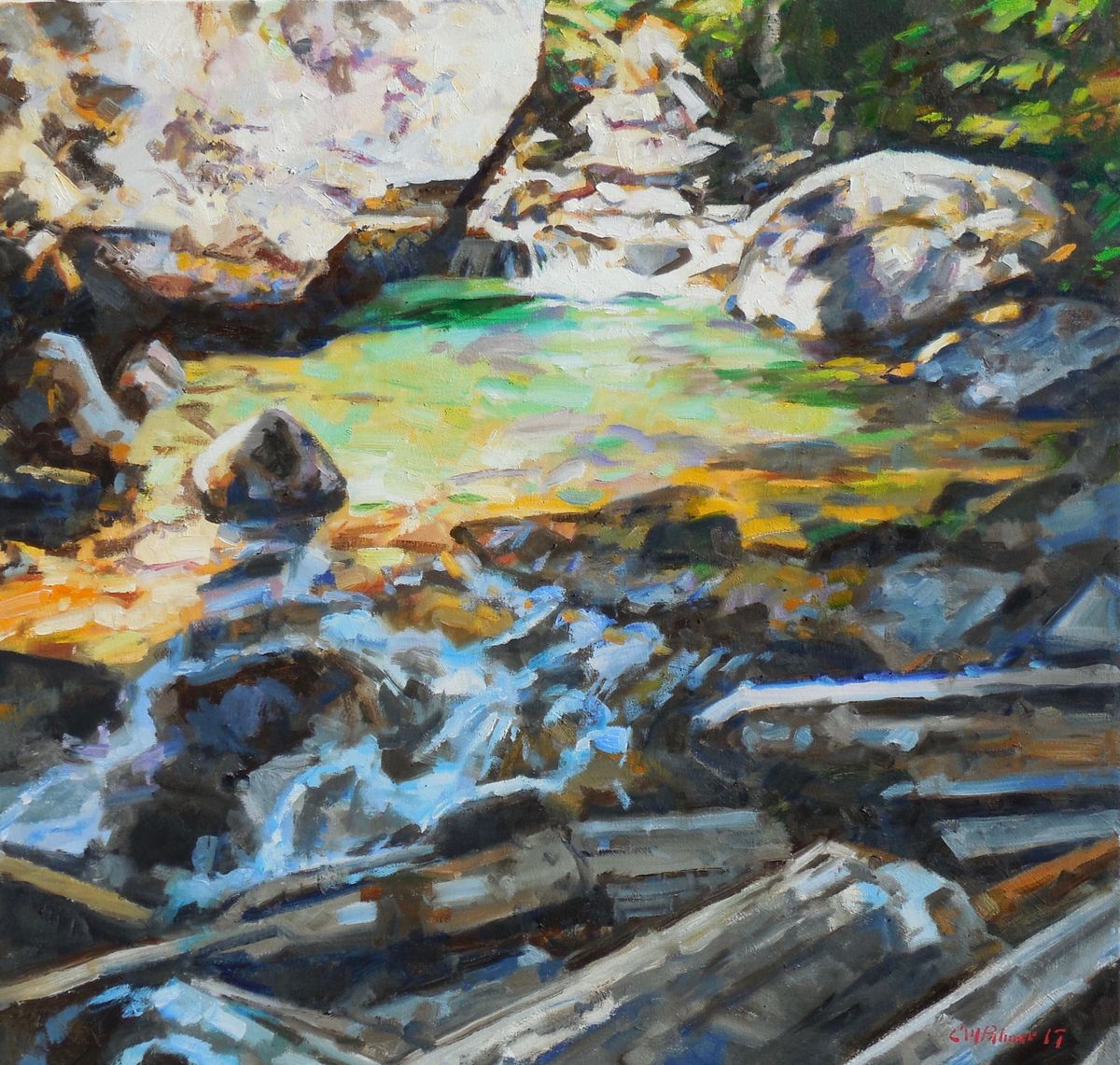The image showcases a vibrant, impressionist-style painting of a river flowing through a forest scene. The river, featuring a mix of green, yellow, and white hues, cascades downwards over rocks and wood-like structures, forming small rapids and a pool in the center, possibly created by natural dams of stones. Prominent in the scene is a large boulder situated at the top left, alongside other rocks that shape the water's tumultuous path, contributing to the white water. Rough, textured brush strokes depict the dynamic movement of the water and the surrounding natural elements. The presence of leaves and distant cascading waterfalls hint at an encompassing forest, with shadows suggesting it is daytime. In the lower right corner, there is a dark red signature, adding an intriguing detail to the vibrant composition.